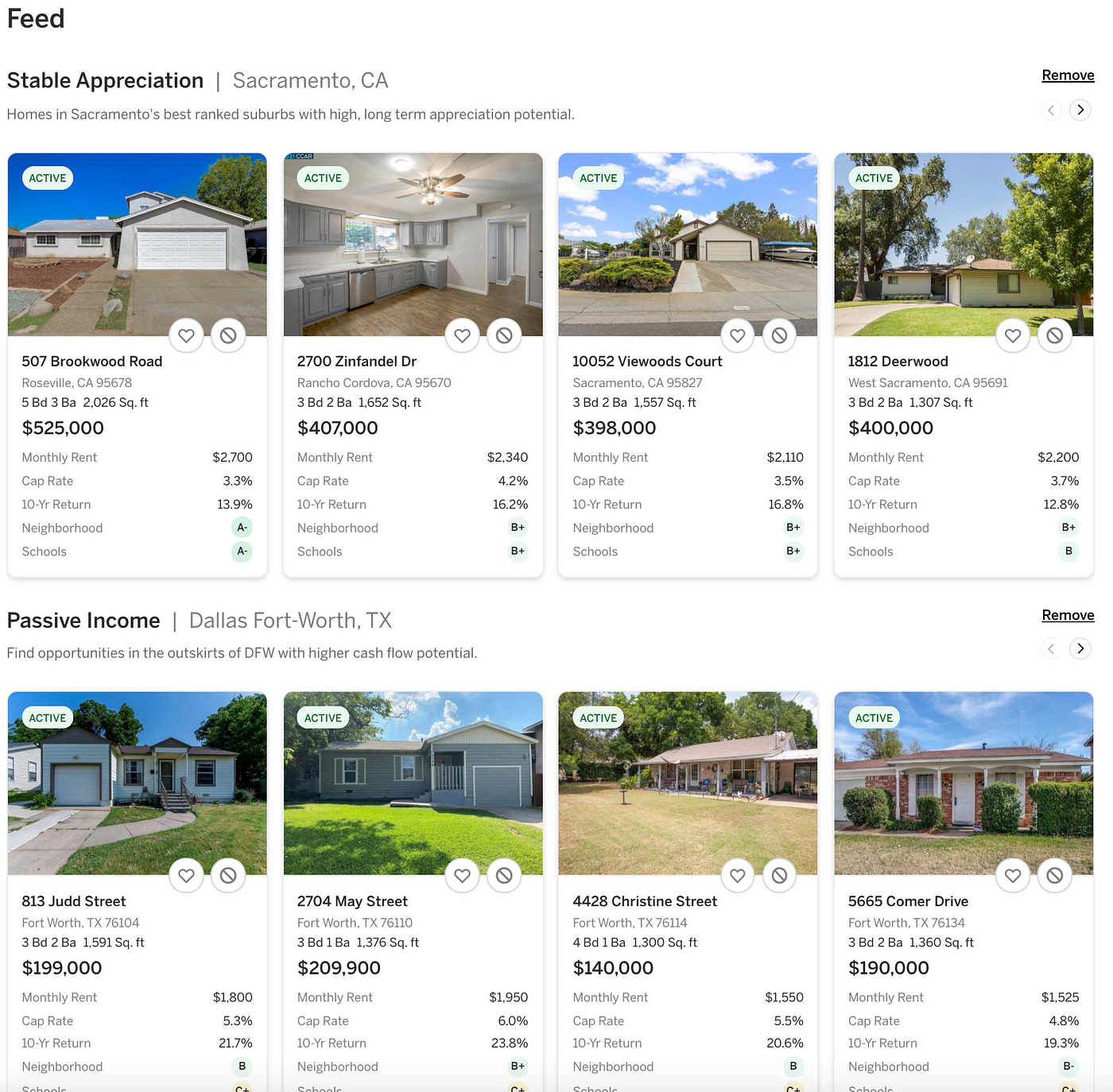This is a comprehensive image showcasing listings of houses for sale in two distinct regions: Sacramento, California, and Dallas-Fort Worth, Texas. Each region displays four different properties with relevant financial details. 

The Sacramento listings emphasize "stable appreciation" and feature property prices ranging from $398,000 to $525,000. Monthly rental estimates for these properties are between $2,110 and $2,700. 

Conversely, the Dallas-Fort Worth listings focus on "passive income," with property prices spanning from $140,000 to $209,900. The estimated monthly rents for these homes are from $1,525 to $1,950. Additional metrics displayed for each property include cap rate, 10-year return, neighborhood score, and school score. 

Overall, the image suggests that potential buyers might be evaluating investment properties, considering both long-term appreciation and rental income opportunities.